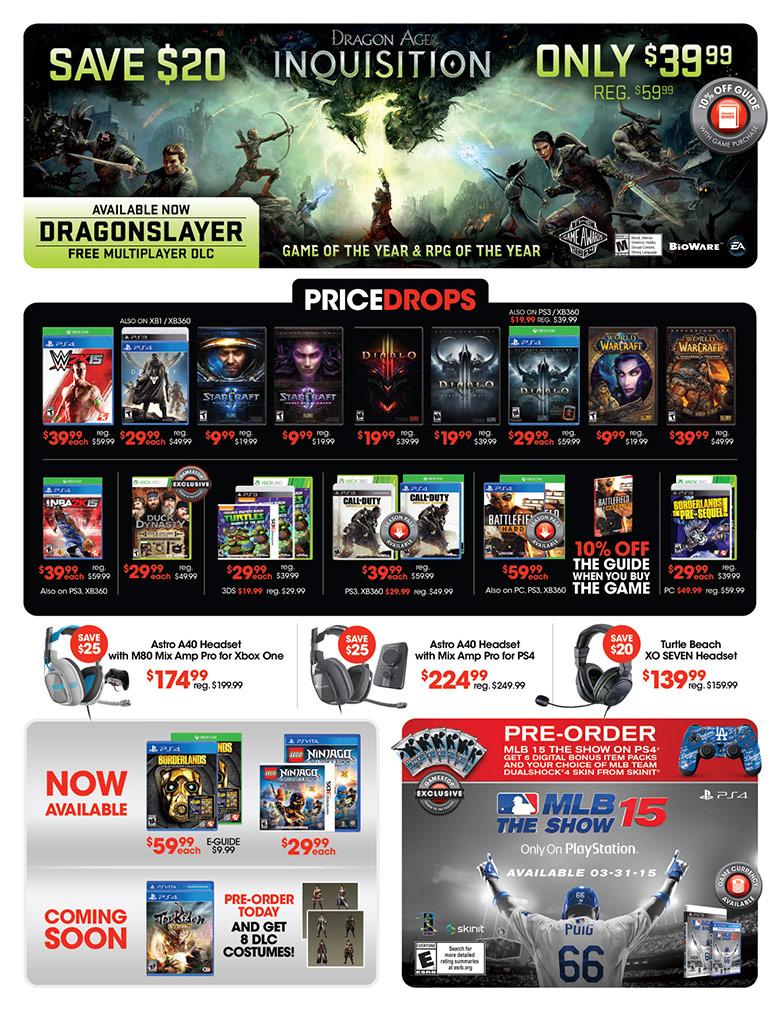This image is a screenshot of a highly dynamic and vibrant website dedicated to computer gaming. At the top, the header prominently features a promotion for "Dragon Age Inquisition," emphasizing a $20 discount, reducing the price to $39.99. Accompanying this banner are vivid game graphics, a mention of the Dragon Slayer multiplayer DLC, and the accolade of being a "Game of the Year RPG."

Below the header, there's a prominent black field highlighting 'Price Drops' for approximately 18-20 games, encompassing various genres such as soccer games, fighting games, and space games. Notably, "StarCraft" and multiple "Diablo" titles are showcased. The old and new prices are displayed in red, typically ranging from $9.99 to $39.99.

Further down, there is a section featuring options for gaming headsets. Three different headsets are displayed, each offering a $25 discount. The prices are $174.99, $224.99, and $139.99 respectively, indicating they are high-quality, premium products.

At the bottom, two additional panels are present. The left panel, titled 'Now Available,' lists new releases such as "Borderlands" and "Ninja Age," priced at $59.99 and $29.99 respectively. The 'Coming Soon' panel hints at upcoming games, though specific titles are unreadable. On the right-hand side, a section dedicated to "MLB The Show 15" is shown, featuring an image of Puig with a stadium backdrop, alongside various controllers and gaming accessories.

Overall, the website offers a robust catalog of games and gaming peripherals, though the specific company behind the site is not identified in the image.